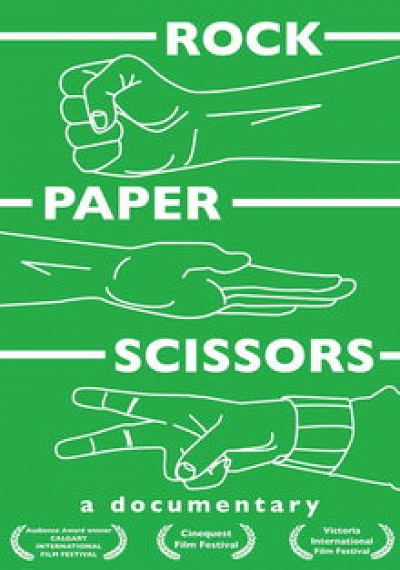The poster for the documentary "Rock, Paper, Scissors" features a medium green background reminiscent of a darker shade of Kermit the Frog. At the very top, in bold, all-capitals white font, is the word "ROCK." Directly below this is a white line-drawing illustration of a fist, symbolizing "rock" in the game. Further down the poster, the word "PAPER" also appears in all-capitals white font, accompanied by a line drawing of a hand held flat, representing "paper." Beneath this, the word "SCISSORS" is displayed in the same white font, with an accompanying illustration of a hand configured to mimic the appearance of scissors. Below the sequence of game symbols, the text "A DOCUMENTARY" is presented in white font. At the bottom of the poster, a text block lists three film festivals that have featured the documentary.